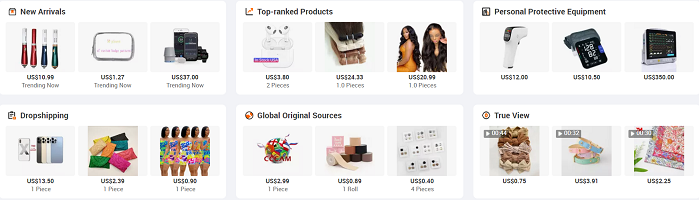The image displays six distinct white boxes, arranged in two rows of three, separated by thick gray lines. Each box contains a title in the upper left-hand corner and three items, complete with descriptions and prices.

Starting from the top left, the first box is labeled "New Arrivals," accompanied by an icon resembling a box with something red inside it. Within this box, there are four objects priced at $10.99, a rectangular object for $1.27, and some black items priced at $37. The phrase "Trending Now" appears, though it is somewhat unclear.

Moving to the right, the second box is titled "Top Ranked Products" and features an icon of a right angle with an arrow emerging from the corner. The first item depicted resembles a hippo and is priced at $3.80. The next item is a mixed color (black, white, and tan) object, priced at $24.33. The final item in this box shows an image of two women with very long hair, priced at $26.99 for one piece.

The third box, positioned next to the second one, is labeled "Personal Protective Equipment." The specific details of the items in this box are not provided in the description.

Overall, the detailed layout and organization of the products facilitate easy browsing, with a clear emphasis on categories and item specifications.